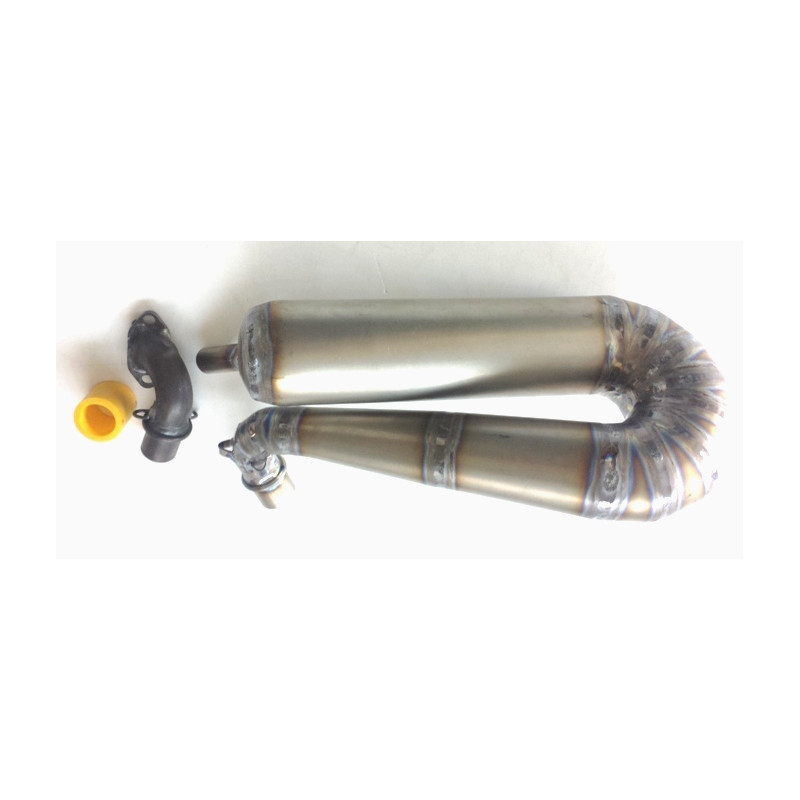This detailed photograph showcases three objects displayed on a white background. On the left side of the image, there is a small yellow cylindrical tube, likely made of plastic. Positioned to its right is a short black metal tube that bends smoothly at approximately a 45-degree angle. Dominating the right three-quarters of the image, a large, intricately curved metallic object takes center stage. This primary object starts with a horizontal tube at the top, which transitions into a 180-degree downward U-shaped curve adorned with colorful metallic bands. The tube then extends leftward beneath the upper section, continuing in a shiny metallic material, and further curves downward at a 90-degree angle toward a metallic cap at the bottom. The overall arrangement suggests a utilitarian purpose, possibly related to plumbing or another mechanical application, although the exact function of these components remains uncertain.